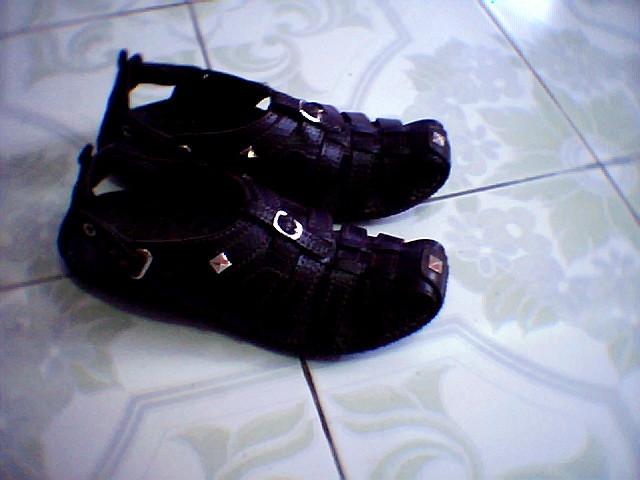The image depicts a pair of small black shoes designed like Roman sandals with closed covered toes, suitable for a young child, possibly around four years old. The shoes are placed side by side on a vinyl floor with a white and pale green flowery tile pattern, interspersed with muted yellows, golds, and light gray shapes. Each shoe features a silvery metal buckle and a design comprising a long strip running from the toe to the ankle, along with multiple strips crossing the foot and an additional strip for securing around the heel. Notably, there are small silver and red emblems on the sides near the buckles, adding a distinctive touch to their appearance.